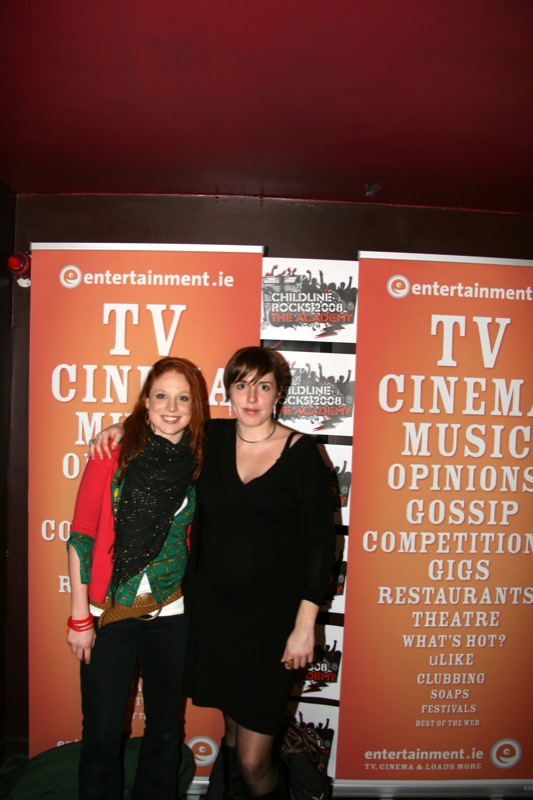This color photograph captures two women posing closely together in an indoor setting likely related to entertainment or a conference. The woman on the left has long red hair and dons a colorful ensemble consisting of a blue jacket over a green vest, accessorized with a black scarf, paired with black pants. The woman on the right, who has short brown hair, is wearing a short black dress and has her right arm affectionately draped over the shoulder of the woman next to her. Both women are standing in front of two tall orange signs emblazoned with white text listing various entertainment-related words such as TV, Cinema, Music, Opinions, Gossip, Competition, Gigs, Restaurants, Theater, What's Hot, You Like, Clubbing, Soaps, and Festivals. At the bottom of the signs, the website entertainment.ie is prominently displayed, along with a central sign indicating "Childline Rocks 2008 Academy,” all contributing to a vibrant, entertainment-centric atmosphere.